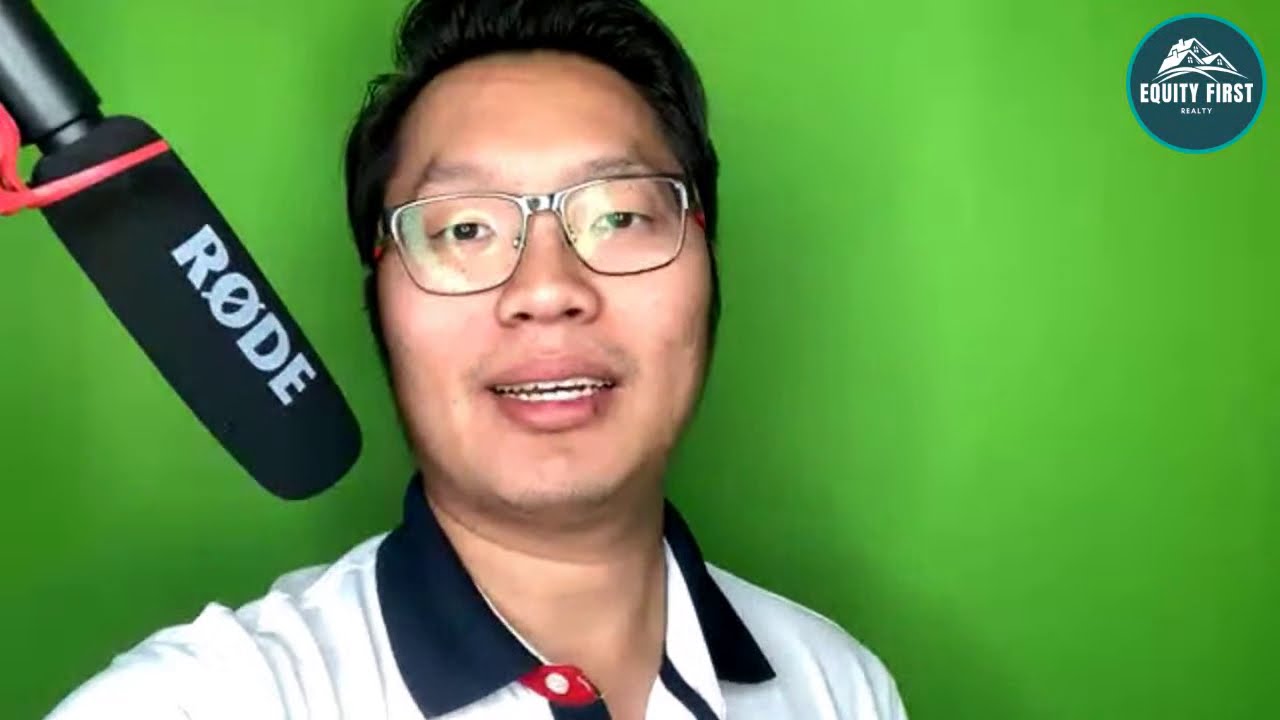This image is a detailed screen grab from a video featuring an Asian man in his 30s, appearing clean-shaven with short black hair and wearing glasses. His face, along with his upper shoulders, is visible in this close-up shot. He is dressed in a white polo shirt with a blue collar. The man stands in front of a green screen and is positioned with a Rode shotgun microphone, indicating he might be delivering a talk or presentation. In the upper right corner of the screen, there is a logo that reads "Equity First Realty," displayed within a green circle that features an illustration of three rooftops. The man's mouth is open, likely captured mid-sentence, and the reflection of a ring light can be seen on his glasses, further hinting at a recording setup suitable for professional video content.